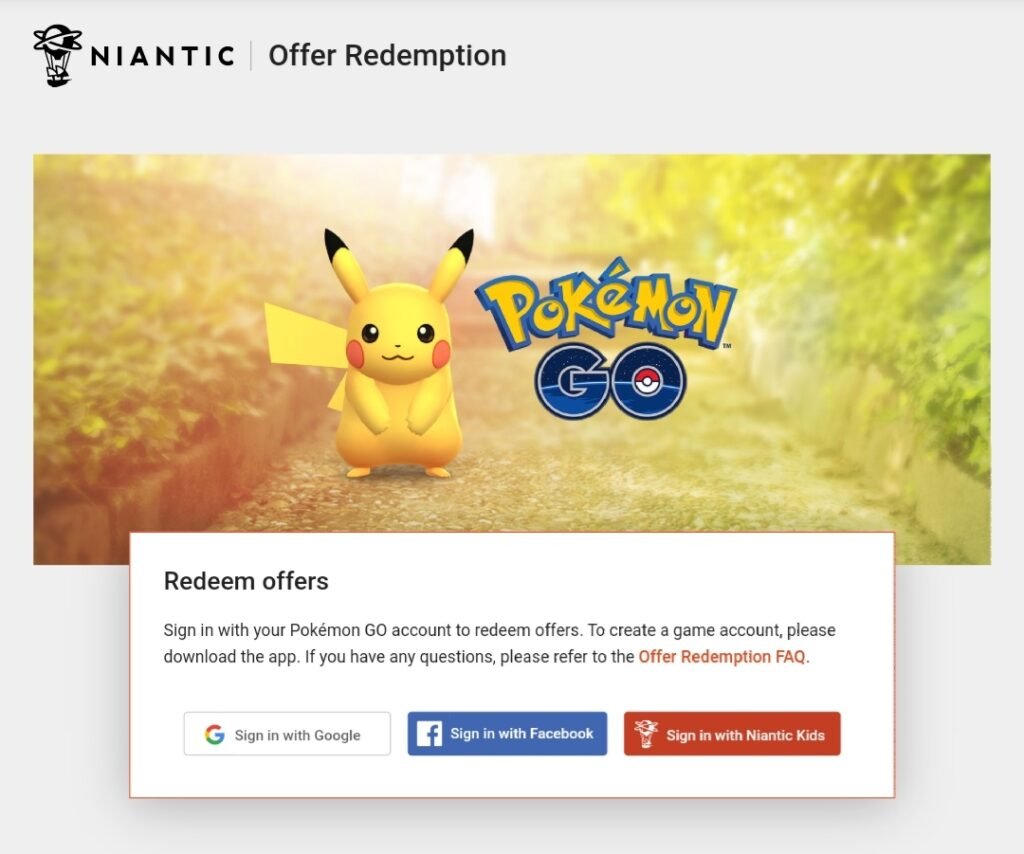The top left corner of the image prominently features the Niantic logo, associated with the popular game Pokémon Go. The centerpiece of the image depicts an airship with a large sphere at the top and a ship at the bottom, adding an adventurous atmosphere. The background has dynamic lighting that transitions smoothly from left to right, creating a vibrant pathway. In the foreground, a Pikachu, with its distinctive yellow body and red cheeks, is staring directly at the viewer, adding a familiar and inviting element.

A prominently placed square invites users to "Redeem Offers." The text within the square instructs users to sign in with their Pokémon Go account to redeem various offers. It also provides a brief guide for new users, suggesting they download the app to create a game account, and directs any inquiries to the "Offer of Redemption" tab. Below this, options to sign in with Google, Facebook, or Niantic Kids are presented, with each button styled distinctively; the Niantic Kids option is highlighted in red.

The image is framed with red borders at the top, which highlights the word "Pokémon", complete with the signature accent over the "E". "Go" is depicted with a blue planet, symbolizing Earth, cleverly designed to resemble a Pokéball. Pikachu is standing on a photorealistic terrain, contrasting with its cartoonish, digitally-drawn appearance. Overall, this image appears to be an advertisement for a Pokémon Go redemption website, offering various ways to sign in and redeem special offers.